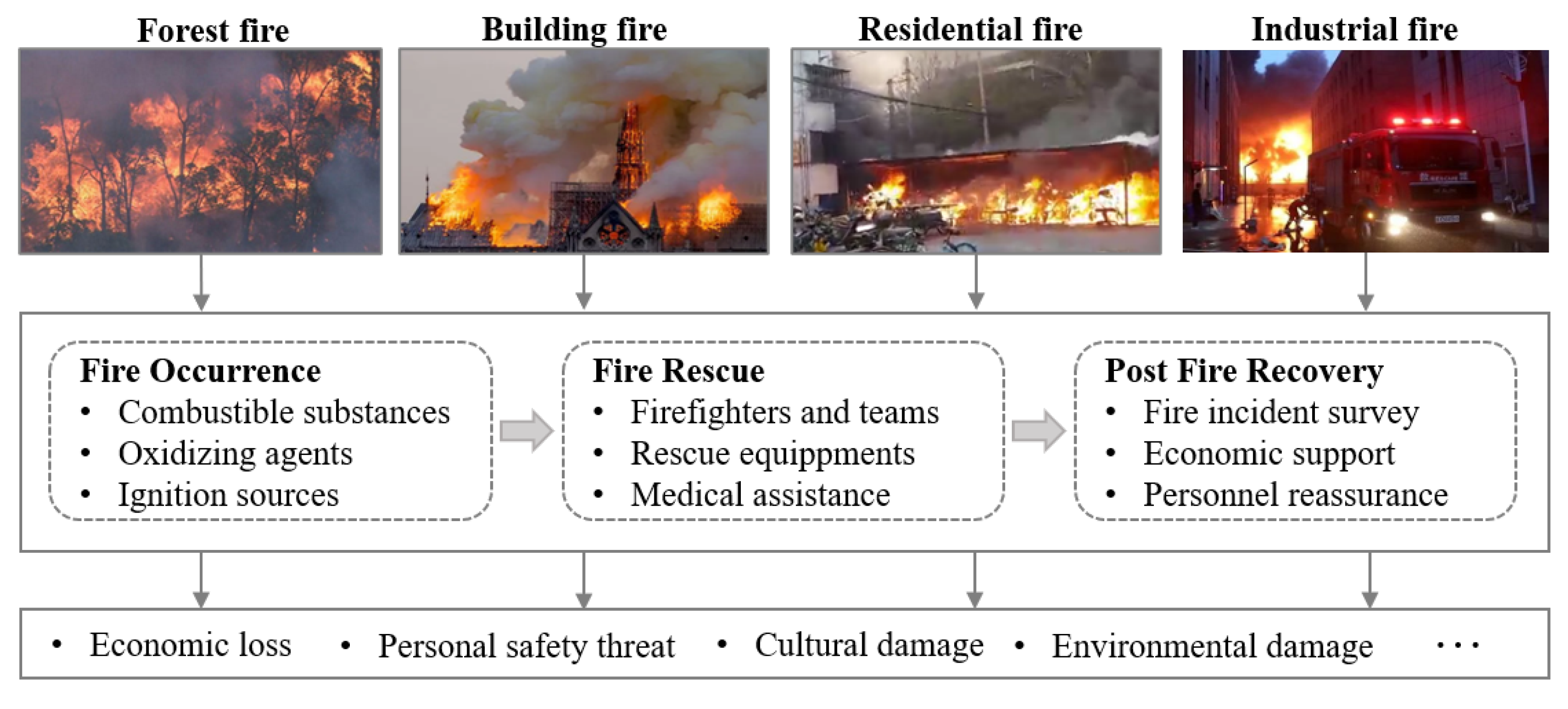The image is a detailed flow chart depicting various fire types—forest fire, building fire, residential fire, and industrial fire—each represented with vivid images showcasing severe flames and dense smoke. Each fire type is categorized under "Fire Occurrence" with details about combustible substances, oxidizing agents, and ignition sources. Arrows guide the flow to "Fire Rescue," highlighting firefighting teams, rescue equipment, and medical assistance. Another arrow leads to "Post Fire Recovery," which includes fire incident surveys, economic support, and personnel reassurance. At the bottom, additional arrows point to specific consequences: economic loss, personal safety threats, cultural damage, and environmental damage. Overall, the chart illustrates the comprehensive impact and management stages of different fire types.